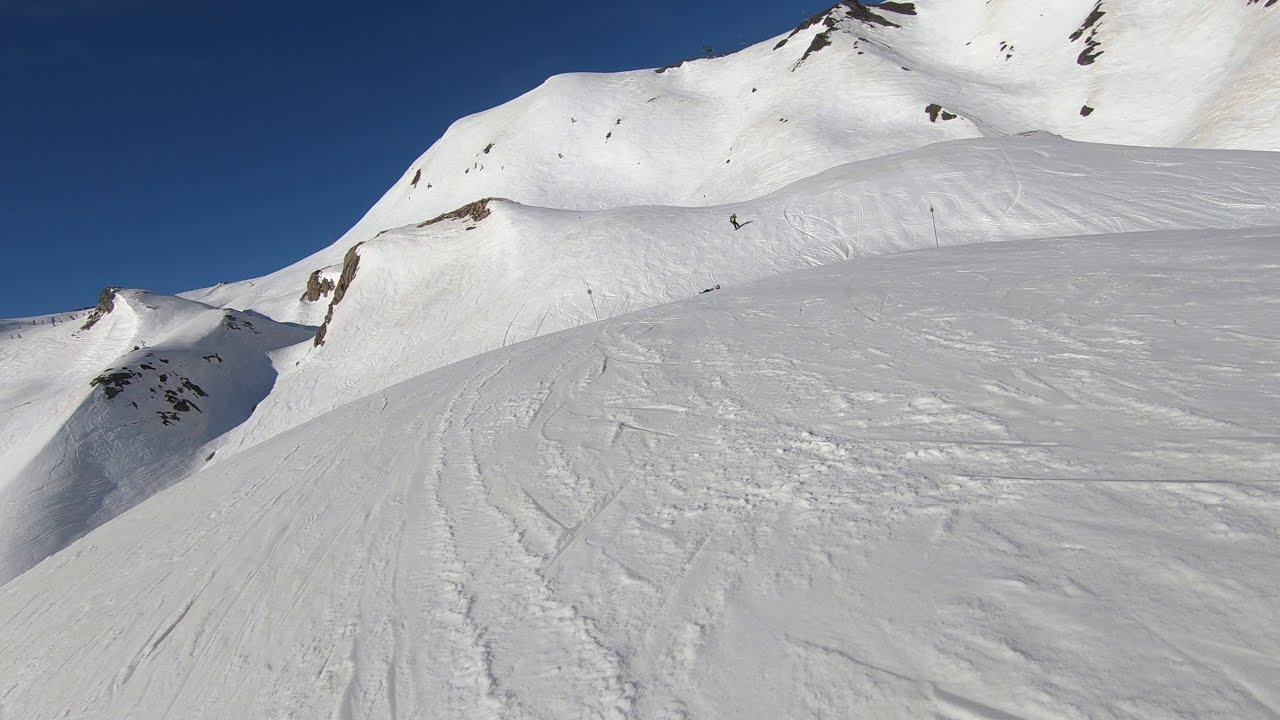The image captures a snow-covered mountainside under a deep, rich blue sky, possibly just before nightfall. The snow is arranged in three distinct tiers: the foreground features a smooth, curved surface; the middle tier is wider but interspersed with rocks; and the background tier is considerably rockier. Tracks from skis and snowboards are scattered across the snow, suggesting recent activity. In the middle tier, there appears to be a tiny person, likely a snowboarder, possibly standing by a ski pole embedded in the ground. There might be another person lying in the snow, hinting at the possibility of the snowboarder joining or assisting them. Despite the presence of these individuals, there is an overwhelming sense of isolation as no other people or wildlife are visible. The snow glistens brightly, creating a stark contrast with the dark, exposed rocks and the vivid blue sky.